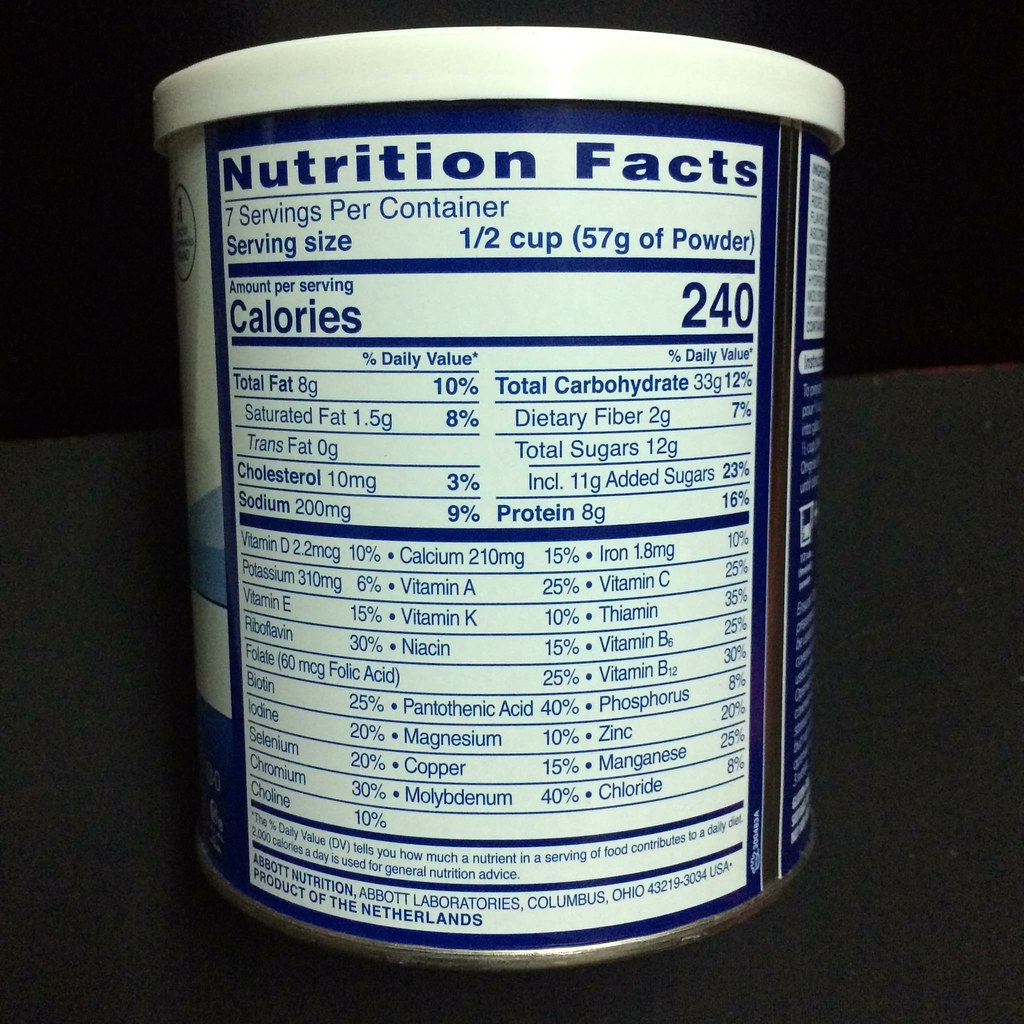This image showcases a cylindrical container, primarily adorned in blue and white hues. The container features a round, white lid and is placed against a predominantly black backdrop with a gray surface beneath it, likely resembling a table. The label, detailed in blue font with white backgrounds, prominently displays "Nutrition Facts" and includes information such as "7 servings per container" and "serving size 1½ cups of powder." Although the specific type of powder is not discernible from the visible side of the label, it is noted to be a product of the Netherlands. The label’s design incorporates a mix of dark blue and light blue, providing a sleek, modern aesthetic.